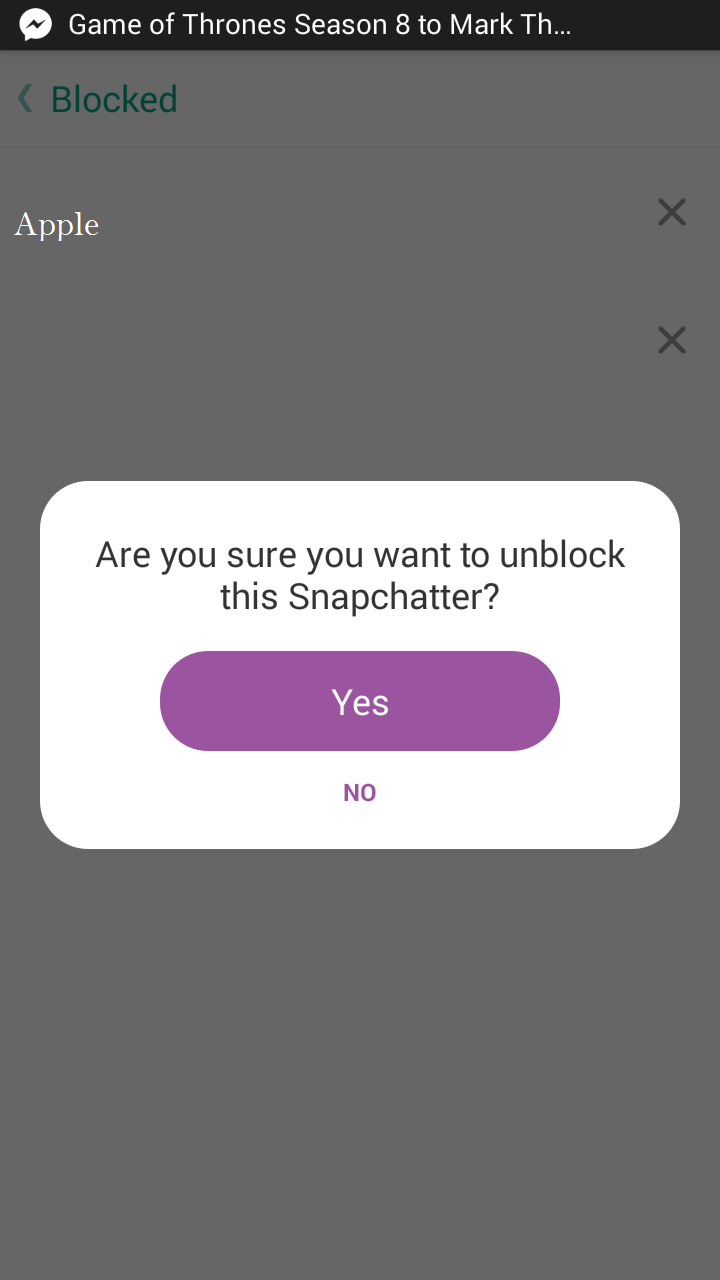A snapshot of a screen displaying a basic interface for watching "Game of Thrones" Season 8. At the top, a narrow black banner shows the title "Game of Thrones Season 8" in small, white text. The background is a faded gray. Below the title, in green text, are the words "Black" underneath "Game of Thrones." Adjacent to this text is a left-pointing arrow. Below the title are the words "Apple" in white text, accompanied by an 'X' to close the window, followed by another 'X' with no corresponding text. A white dialog box has popped up, posing the question, "Are you sure you want to block this Snapchatter?" with options "Yes" and "No." The currently highlighted option is "Yes," shown with a purple tab. Overall, the screen is simplistic with predominantly white lettering and minimal graphics, making for a rather unengaging visual experience compared to the epic visuals typically associated with the series.